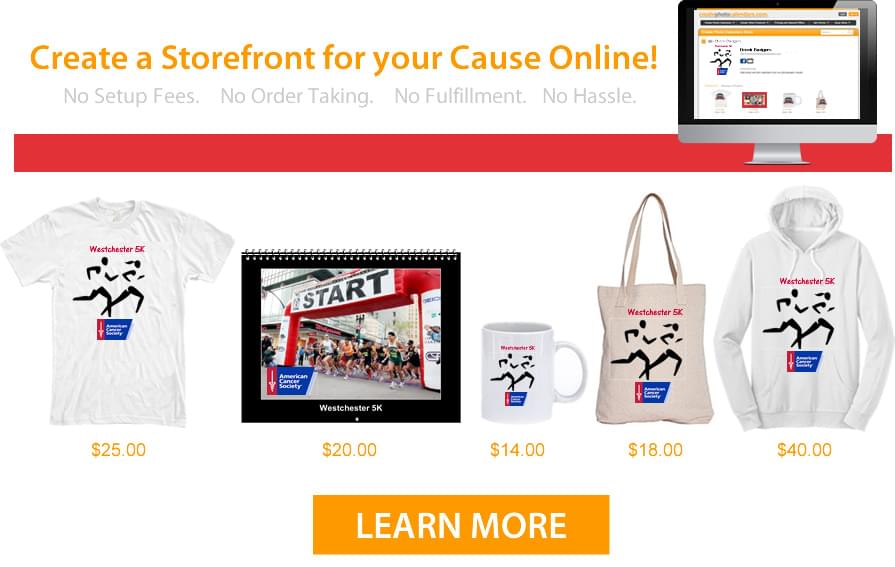This image is a detailed screenshot from a web page promoting an online storefront creation service. At the very top, set against a white background, bold gold-colored text enthusiastically proclaims "Create a storefront for your cause online!" Beneath this, a gray font advertises several key selling points: "No setup fees, no order taking, no fulfillment, no hassle." Adjacent to this text on the right is a smaller screenshot, presumably displaying an example online store; however, the details are indistinct. The visible products appear to include a mug and a t-shirt, while the identities of the other two items are unclear.

Below these elements, a border in a warm brick red hue spans the width of the page. Moving further down, the page showcases various products available for customization with company or organizational logos. From left to right, there is a t-shirt illustrated with a design that suggests participation in an event, such as a road race or marathon; this example features "Westchester 5k" alongside a schematic depiction of two runners. To the right of the t-shirt is a calendar, likely using a photograph from the race's starting line. Next in line is a white mug adorned with the same design seen on the t-shirt, followed by a tote bag and a white hoodie, both featuring the identical running-themed image.

At the very bottom of the image, there is a gold-colored rectangle with white text that invites further exploration with a call to action: "Learn More."